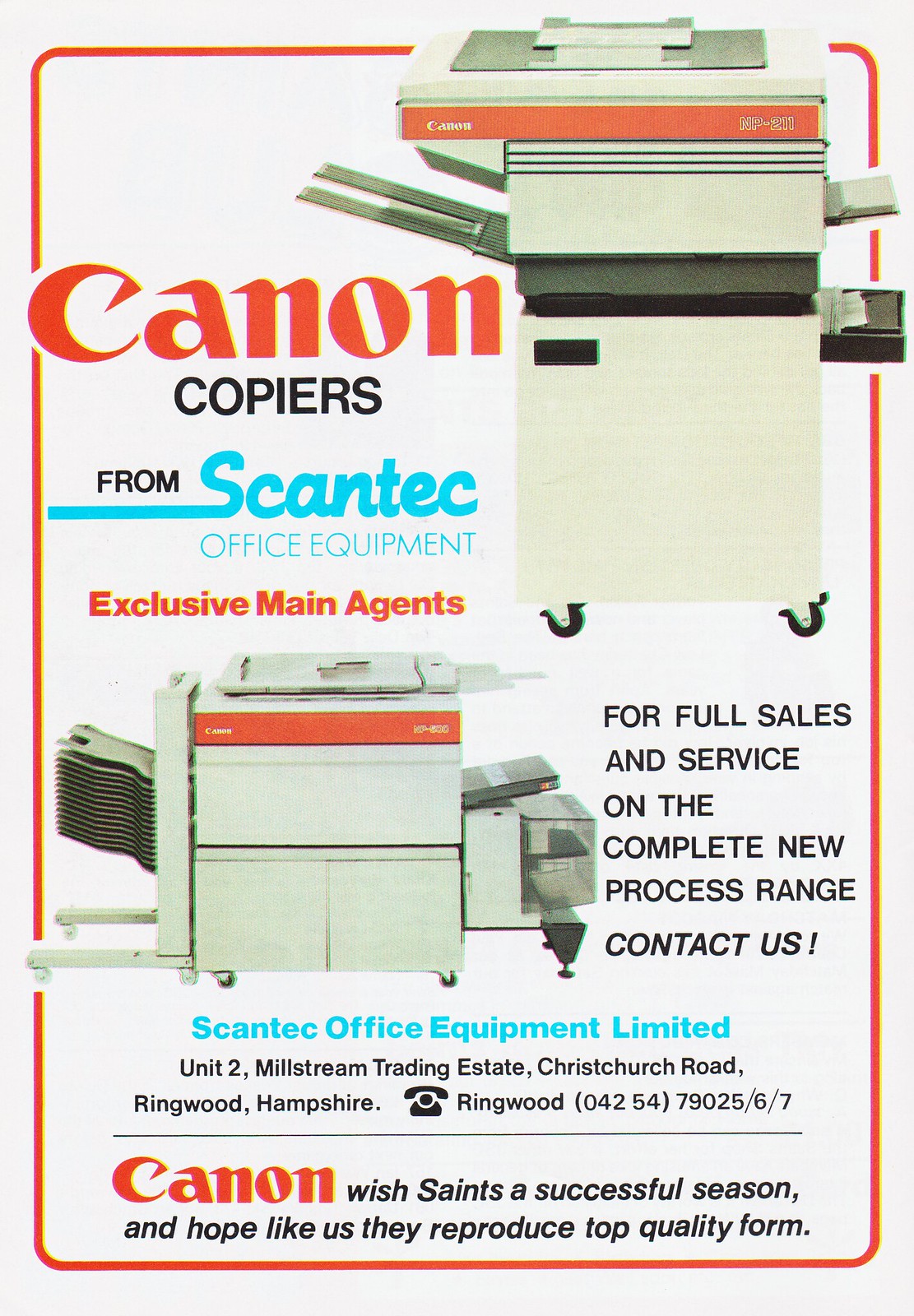This Canon copier advertisement is set indoors and features a clean, graphic design with a prominent orange border. The ad is presented in a rectangular, portrait layout and showcases two images of Canon copiers on wheels. The first image, at the top, is of a white, boxy copier with the text "Canon copiers" to its left. "Canon" is written in orange, while "copiers" is in black. Below this, the text "from Scantech Office Equipment" appears in light blue, followed by "Exclusive Main Agents" in orange.

A wider copier with multiple compartments for holding documents is featured in a photo beneath the first. Next to this image, black text reads, "For full sales and service on the complete new process range, contact us." Below this, in blue, "Scantech Office Equipment Limited" is displayed. Further down, the text continues in black: "Unit 2 Millstream Trading Estate, Christchurch Road, Ringwood, Hampshire. Ringwood 04254 79025/6/7."

The advertisement concludes with a goodwill message from Canon: "Canon wish Saints a successful season and hope, like us, they reproduce top quality form." The design integrates elements of both modern and vintage aesthetics, capturing the viewer's attention with its bold colors and comprehensive information.